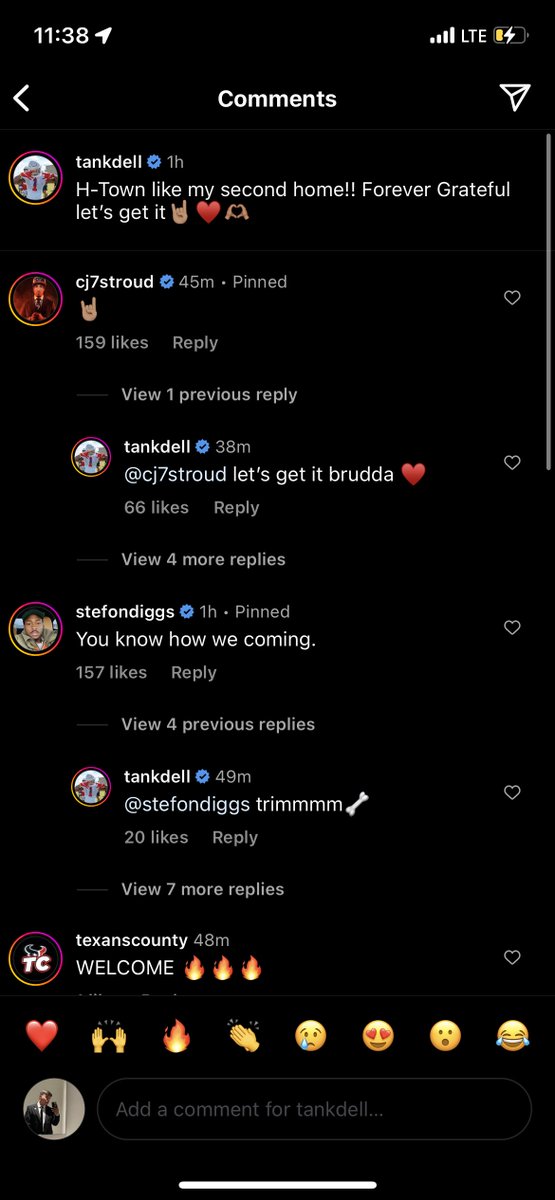### Caption:

A screenshot of an Instagram comment thread displayed in dark mode, where the background is black and the comments are highlighted in white. The comment thread features a sense of camaraderie and excitement among the users. 

1. **Tankdel** initiates the thread with a heartfelt post: "Each town like my second home, forever grateful, let's get it," enhanced with emojis that emphasize his passion and gratitude.
2. A user responds with just an emoji, showing silent approval or reaction, and Tankdel follows up with an enthusiastic reply: "Let's get it, Brudda," capped with a red heart emoji to express affection and camaraderie.
3. Another user comments, "You know how we coming," to which the thread sees various replies, including from the original user, Tankdel, affirming with "Trim," punctuated by a bone emoji.
4. **Texans County** joins the thread with a warm greeting, "Welcome," adorned with three fire emojis that symbolize excitement and energy.
5. At the bottom of the screenshot, options to add another comment and a list of suggested emojis for quick responses are visible, highlighting the interactive aspect of the platform.

At the top of the screenshot, there are navigation options to either go back or send the comment thread, reminding the viewer of Instagram's user interface features. The vibrant interaction among users showcases the shared sense of community and enthusiasm within the thread.